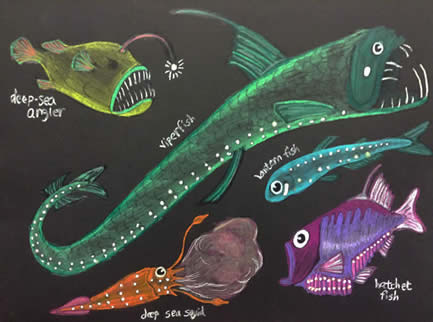The image is a detailed, colorful drawing of deep-sea creatures set against a black background, arranged within a rectangle. At the center, there's a yellow deep-sea angler with sharp, white teeth and a glowing light on top of its head, exuding a shocked or angry expression. Beside it, the long green viperfish also shows off big, menacing teeth, giving it a similar fierce look. Below them, roaming through the depths, is a blue lanternfish adorned with white spots, and underneath that, a purple hatchetfish resembling the shape of a tilapia. Completing the scene is an orange deep-sea squid releasing ink. All the creatures have striking white highlights and eyeballs, adding to their vivid portrayal in the artwork.